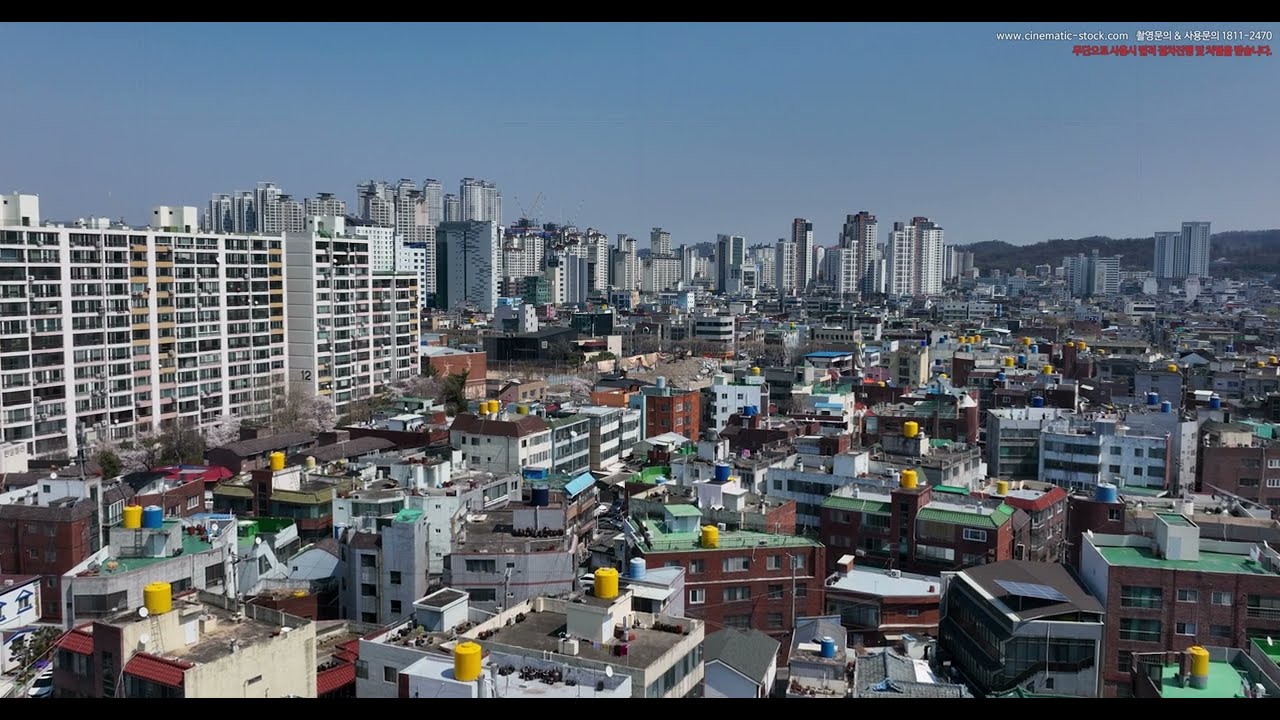The image portrays a densely packed industrial metropolis with a varied cityscape. In the foreground, several buildings, towering two to four stories high, dominate the scene. These structures, closely packed with little to no visible streets, sport bright yellow smokestacks on their rooftops and are predominantly brown or red brick. Interspersed among them are some white buildings with numerous windows, likely serving as businesses. To the left, a prominent 15-story apartment complex stands out, its balconies clearly visible. Directly behind this foreground cluster rises a row of massive skyscrapers that form a striking city skyline against the bright blue sky. The background is a continuous expanse of urban sprawl marked by more buildings and green-roofed structures. Notably, on the upper right corner of the image, there is text in white and red, contributing to the overall bustling and industrial character of the city.